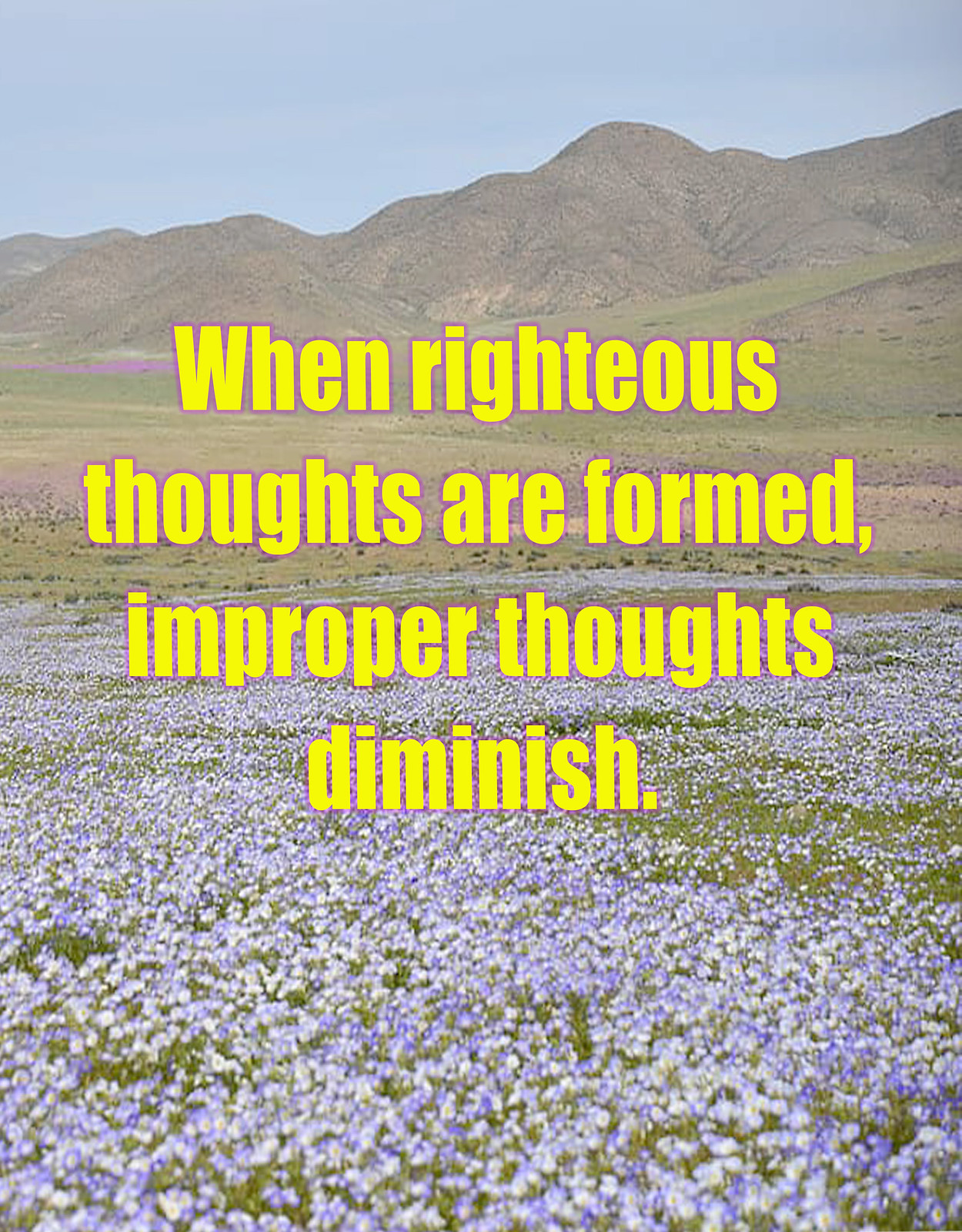The image depicts a vibrant outdoor scene featuring a picturesque flower field with mainly purple blooms interspersed with green grass. The foreground is filled with these purple flowers adorned with bits of white. This colorful meadow transitions into a flat grassland situated below rolling, hilly mountains that dominate the background. The mountains are topped with a light blue sky that's slightly cloudy, giving a hazy atmosphere to the overall scene. Overlaid at the center of the image is an inspirational quote in four lines of yellow text with a light purple shadow. The text reads: "When righteous thoughts are formed, improper thoughts diminish." The image invokes a serene and uplifting natural landscape, emphasizing the effect of positive thinking.